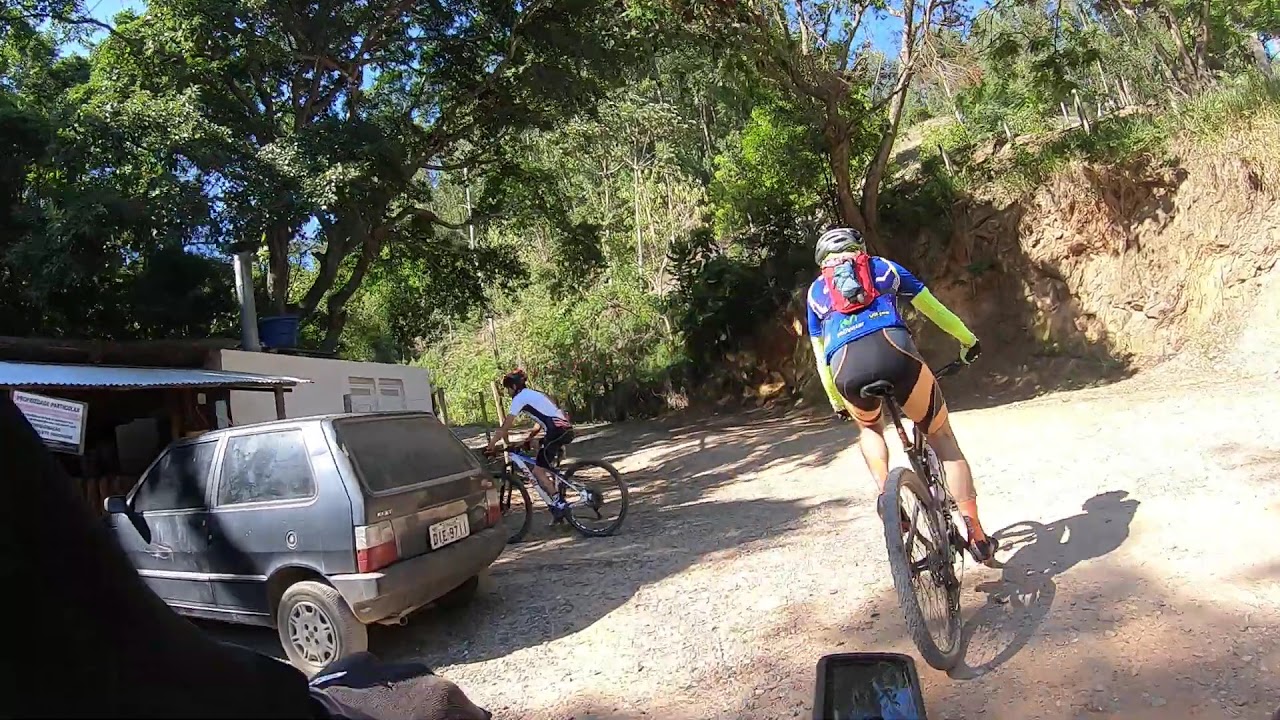This dynamic image, captured from a GoPro perspective, shows two cyclists dressed in full aerodynamic biking gear, including helmets, navigating a dirt or forest path. The rider furthest from the camera, sporting orange and black shorts, orange socks, a green long-sleeve shirt beneath a short-sleeve blue top, leads the descent. To the left, a second cyclist in black shorts and a short-sleeve shirt, also wearing a helmet, makes a left turn. Both cyclists appear focused and determined, indicative of their serious biking intentions. In the background, to the left, an older 90s-era car is parked under a partial roof, suggesting a stop-off point, perhaps at a store. The right side reveals a building alongside a landscape of hilly terrain covered with dense trees and vegetation, framing the scene in a secluded, natural setting, likely somewhere in America. The atmosphere is a mix of adventure and tranquility, capturing a snapshot of an invigorating outdoor pursuit.